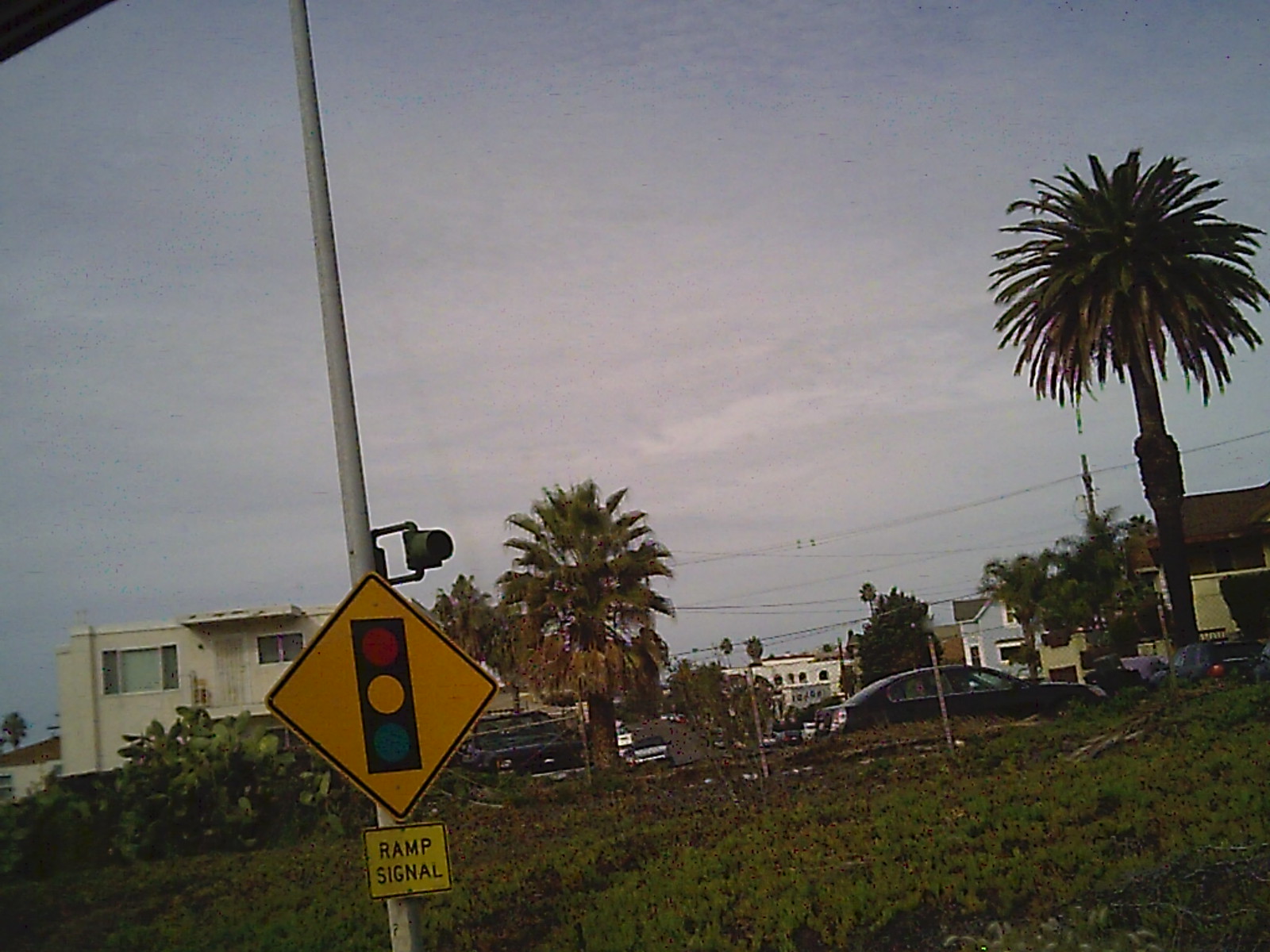This vintage-looking photograph captures a picturesque tropical scene, likely near a beach. Central to the image is a cluster of beach houses with distinct colors and characteristics. In the foreground, there is a white flat-roofed house adorned with a few palm trees and lush greenery, including elfin ears. This house has the appearance of a potential rental property. Adjacent to it on the right are two other houses, one painted a vibrant blue and the other a warm beige. The sky above is a moody grayish-blue, lending an aged feel to the photo. The presence of modern cars in the foreground contrasts with the scene's overall nostalgic aesthetic. Additionally, a large traffic pole topped with a non-flashing light and a "RAMP SIGNAL" sign prominently stands in the foreground, suggesting the proximity of an approaching ramp, possibly leading to a bridge over the water.